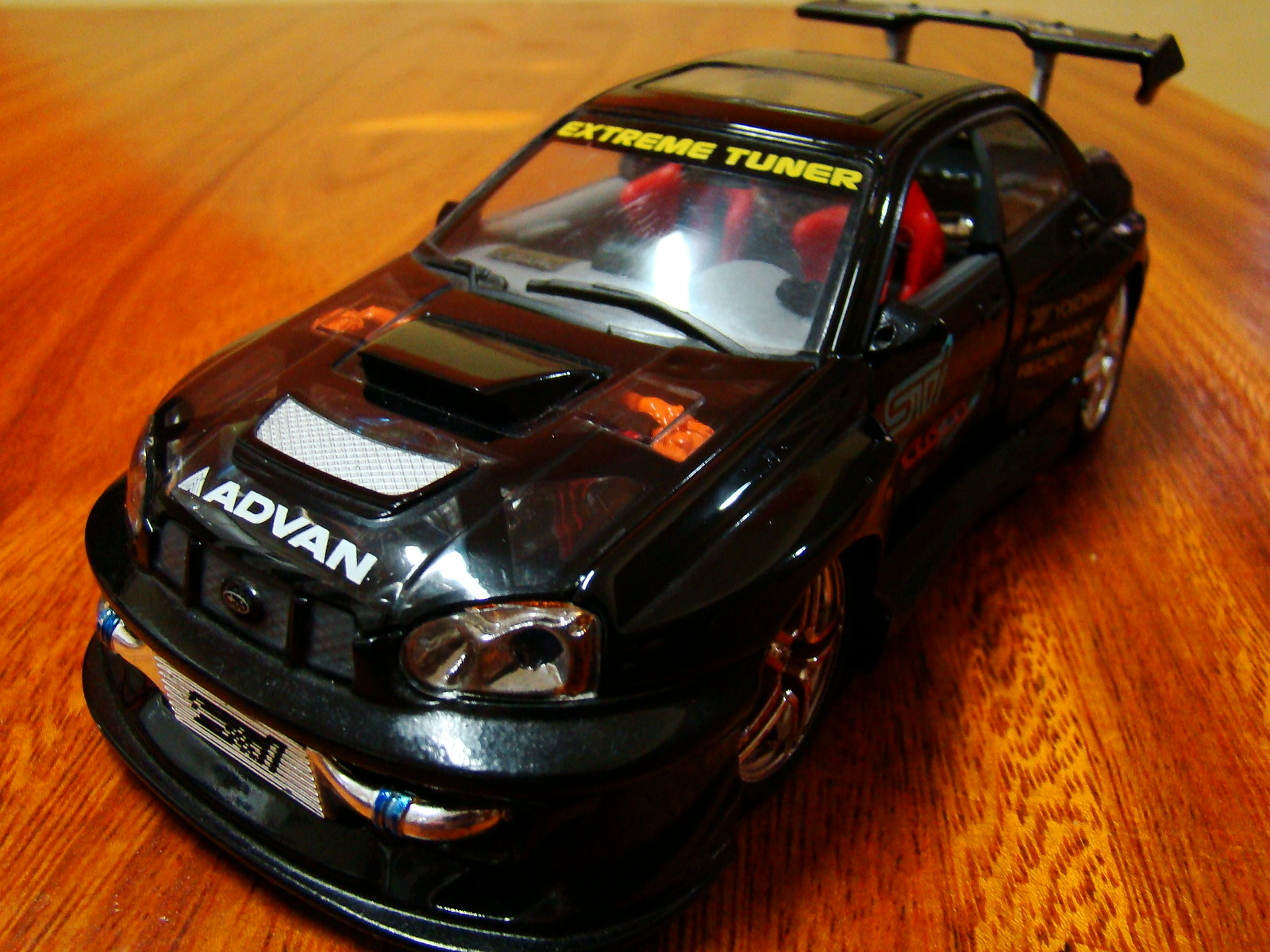The image showcases a highly detailed, photographic portrayal of a black scale model racing car displayed indoors. The car, positioned to face the lower left corner of the frame, is set against a medium brown wooden surface, highlighting the wood's striations with hints of red in the stain. This surface could either be a table or a floor. The model car features vivid red seats and silver hubcaps, accentuated by its sleek, black exterior. Prominently, the top of the windshield bears the phrase "EXTREME TUNER" in yellow, capital letters, while the front hood displays the word "AADVAN" in white lettering. The car also includes a black spoiler at the rear, a sunroof, and small windshield wipers. A notable detail is the presence of a license plate graphic on the front, albeit without any discernible numbers or text. A flash in the photograph creates a glare on the windshield, further emphasizing the car's glossy finish and intricate design elements. In the background, a table with three legs is just visible, adding to the indoor setting's depth and context.